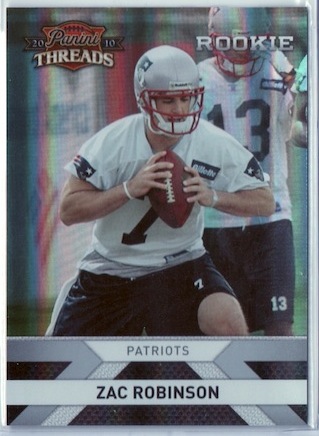This detailed, vertically-oriented trading card from the 2010 Panini Threads collection features a rookie named Zach Robinson, who played for the Patriots. The card prominently displays the word "Rookie" in white text with a black border in the top right corner, while "Panini Threads 2010" is noted in the top left. The main image centers on Robinson, clad in a white football jersey with a bold blue number 7, blue shorts with a smaller number 7, and a silver helmet with a red face guard. Robinson, possibly a quarterback, is depicted with a football in hand and a wristband on both wrists, poised to make a throw on the football field. Behind Robinson, another player wearing a white jersey with a large number 13 and matching blue shorts is visible. The bottom of the card is bordered in silver, displaying the text "Patriots Zach Robinson." The scene includes a mix of red, blue, white, silver, and gray colors, adding to the dynamic and authentic football card design.